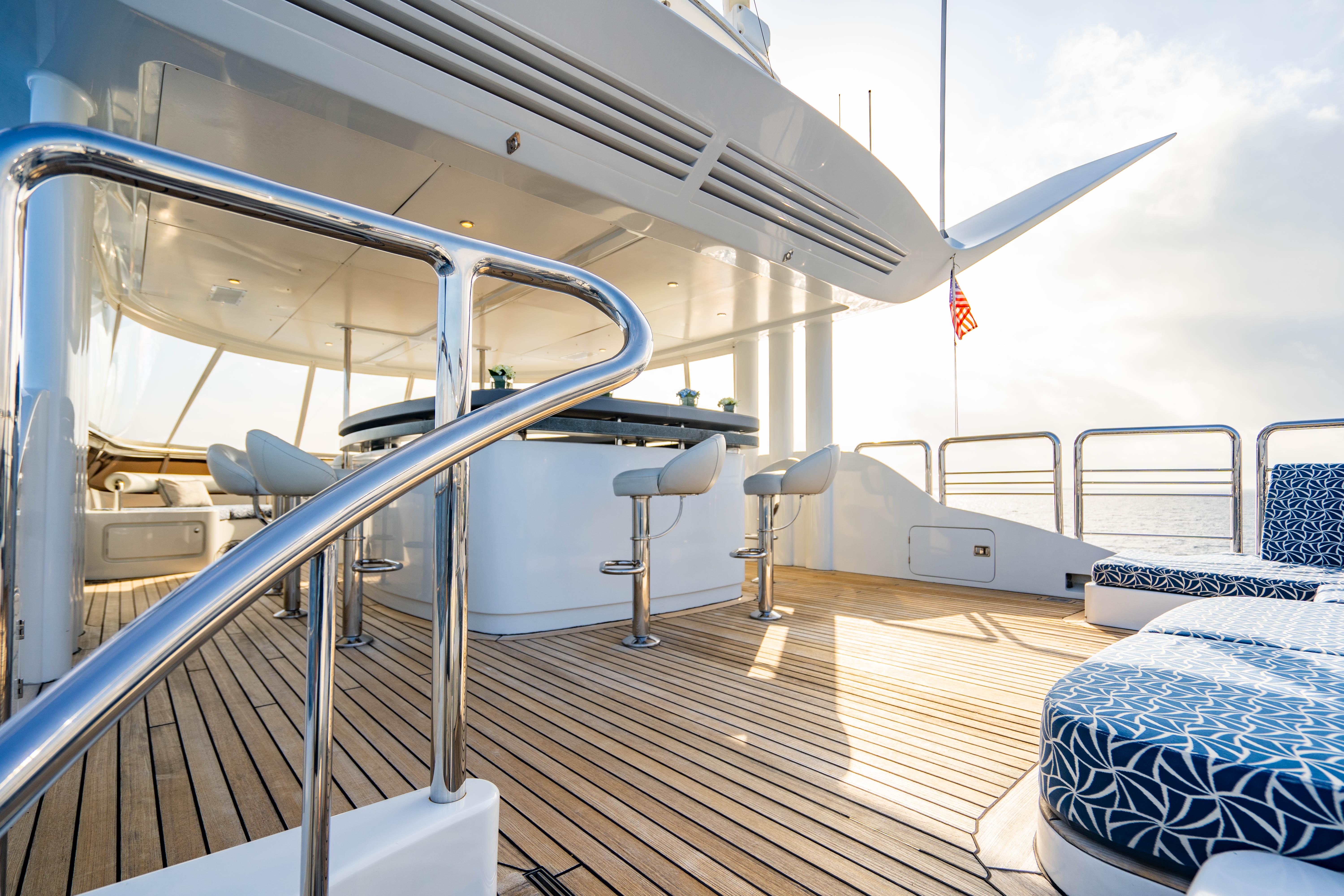The photograph, taken outdoors during the daytime on a yacht, captures a scene bathed in clear blue skies with scattered white clouds in the background. Dominating the center of the image is a square-shaped bar area with sleek white leather stools encircling it. Adjacent to the bar on the right-hand side is an inviting seating area adorned with blue cushions that feature intricate white patterns, set upon a light brown wooden deck. To the left, a large silver metal handrail with vertical posts mounted on a white base confirms the maritime setting, extending diagonally from the lower left before curving back to the left. Above the area, an overhead enclosure forms a shaded roof, indicative of the yacht's upper level. An American flag is visible in the upper right corner of the image. The overall color palette includes shades of blue, white, tan, silver, brown, red, and gray, accentuating the luxurious and tranquil atmosphere of the yacht.